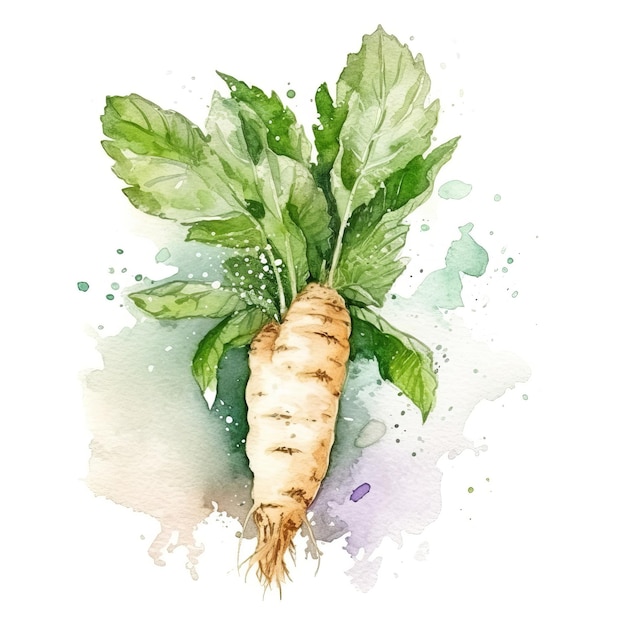This watercolor painting captures an abstract depiction of a root vegetable, primarily resembling a carrot with hints of other root vegetables like turnips or rutabagas. The vegetable starts at a beige root, transitioning through shades of medium brown with small brown divots. It concludes with numerous fine, hairy roots at the tip. The top of the vegetable splits into multiple lobes from which sprout vibrant green stems adorned with lush, varying shades of green leaves, some lighter and some darker. These leaves are expansive, almost equal in size to the vegetable itself, and exhibit intricate veining.

The background is pure white, accentuated by splashes of color. Pale brown dominates the left side, transitioning to shades of green at the center, with bursts of purple and very pale green towards the bottom and top right, respectively. The colorful splatters and splotches surrounding the vegetable give an impression of motion, as though it has just been pulled out of the ground, causing an explosion of hues and droplets. The abstract nature of these splashes further enhances the artwork’s dynamic and lively feel, complementing the central root vegetable.